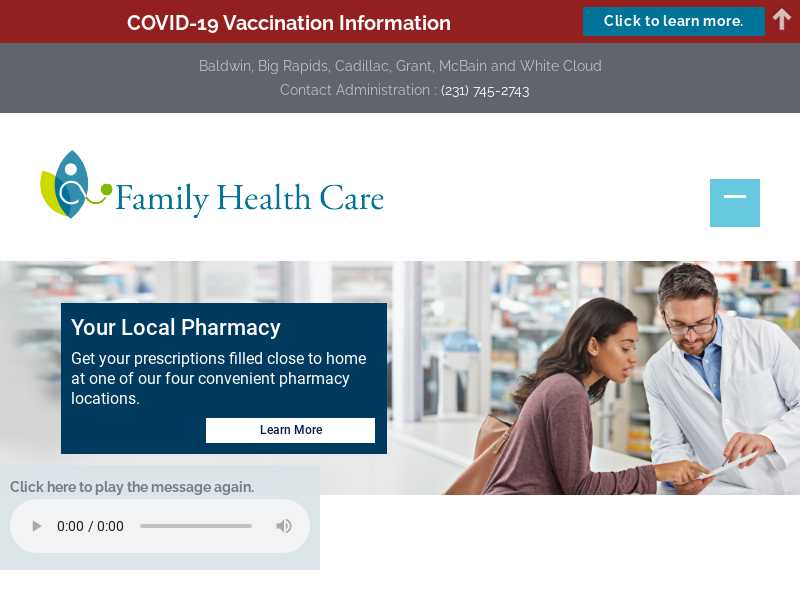**Detailed Description of the Screenshot:**

The screenshot captures a webpage featuring important information about COVID-19 vaccination. At the very top, there is a dark red header with centered white text that reads "COVID-19 Vaccination Information." Adjacent to this text, after some empty space, there is a teal blue button with white text that reads "Click to Learn More." Further to the right on the same red background, there is a white arrow pointing upwards.

Below the red header, another header appears in dark gray with centered white text, displayed over two lines. The first line lists locations: "Baldwin, Big Rapids, Cadillac, Grant, McBain, and White Cloud." The second line provides contact information: "Contact Administration:" followed by a bright white phone number, "231-745-2743."

Underneath this section, there is a white header featuring an abstract logo on the left. The logo comprises blue and green leaf-like shapes with a green stethoscope design extending to the right. Next to the logo, three teal blue words read "Family Health Care." On the far right of this header, after a section of blank space, there is a light blue box with a white minus sign towards the top center of the box.

In the background of the image, a brightly lit white pharmacy is visible. At the bottom right of the image, a counter is seen, with a doctor or pharmacist in a white lab coat and glasses leaning on it from the right. To the left of the pharmacist, a woman in a burgundy brownish shirt with long brown hair, carrying a brown purse, is leaning over the counter, attentively looking at a white piece of paper that the pharmacist is holding. Overlaying this photograph, on the left side of the image, is a dark blue box containing white text.